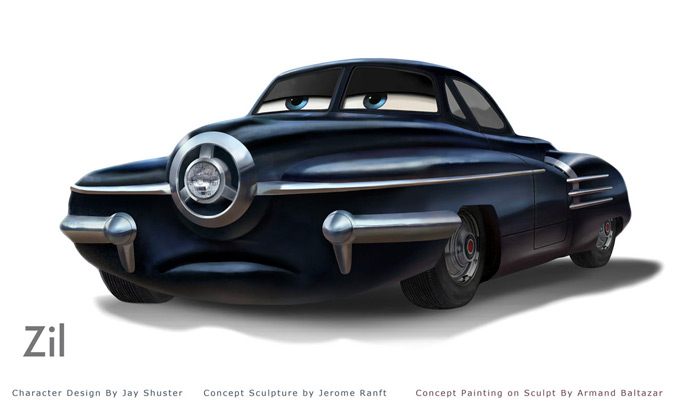This is a horizontally rectangular digital artwork featuring a sleek, black car character design from the movie *Cars*. The image lacks a definitive border or background, emphasizing the character itself. The car, named Zill, has a distinctive 1950s aesthetic, marked by its split windshield that forms its half-closed blue eyes, giving it a tired expression. The front features a prominent round grille with a single headlight in the middle, bordered by chrome detailing that extends towards the doors. Additional large chrome bars adorn the lower sides of the front, accentuating its vintage appeal. The red metallic circle where its nose would be adds a unique touch, and its mouth is closed, integrated into the bumper. Text at the bottom left reads "Zill" in gray letters, and additional text credits the creators: "Character Design by Jay Schuster, Concept Sculpture by Jerome Ranth, and Concept Painting on Sculpt by Armand Baltazar."